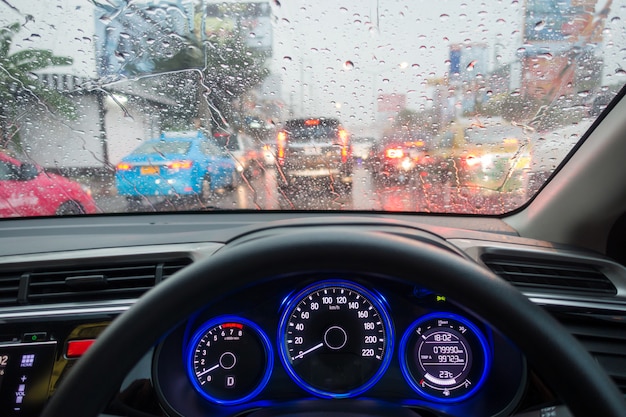This photograph captures an urban scene from inside a likely European car with a right-hand steering wheel. The car's interior looks new, featuring a black steering wheel and a clean dashboard with striking bright blue dials for the speedometer and other metrics. It's a rainy day, evident by the numerous raindrops on the windshield and the wet sheen on the road. The city traffic is heavy, visible through the windshield with several cars ahead, including a yellow car, a black car, a blue car, and a red car, all with their brake lights glowing and reflecting on the wet street. Additional details include a red button and a radio on the left side of the dashboard. In the blurred background, you can spot buildings and faintly discern palm trees. The overall scene offers a detailed glimpse of the car's interior juxtaposed with the rainy, traffic-laden cityscape outside.